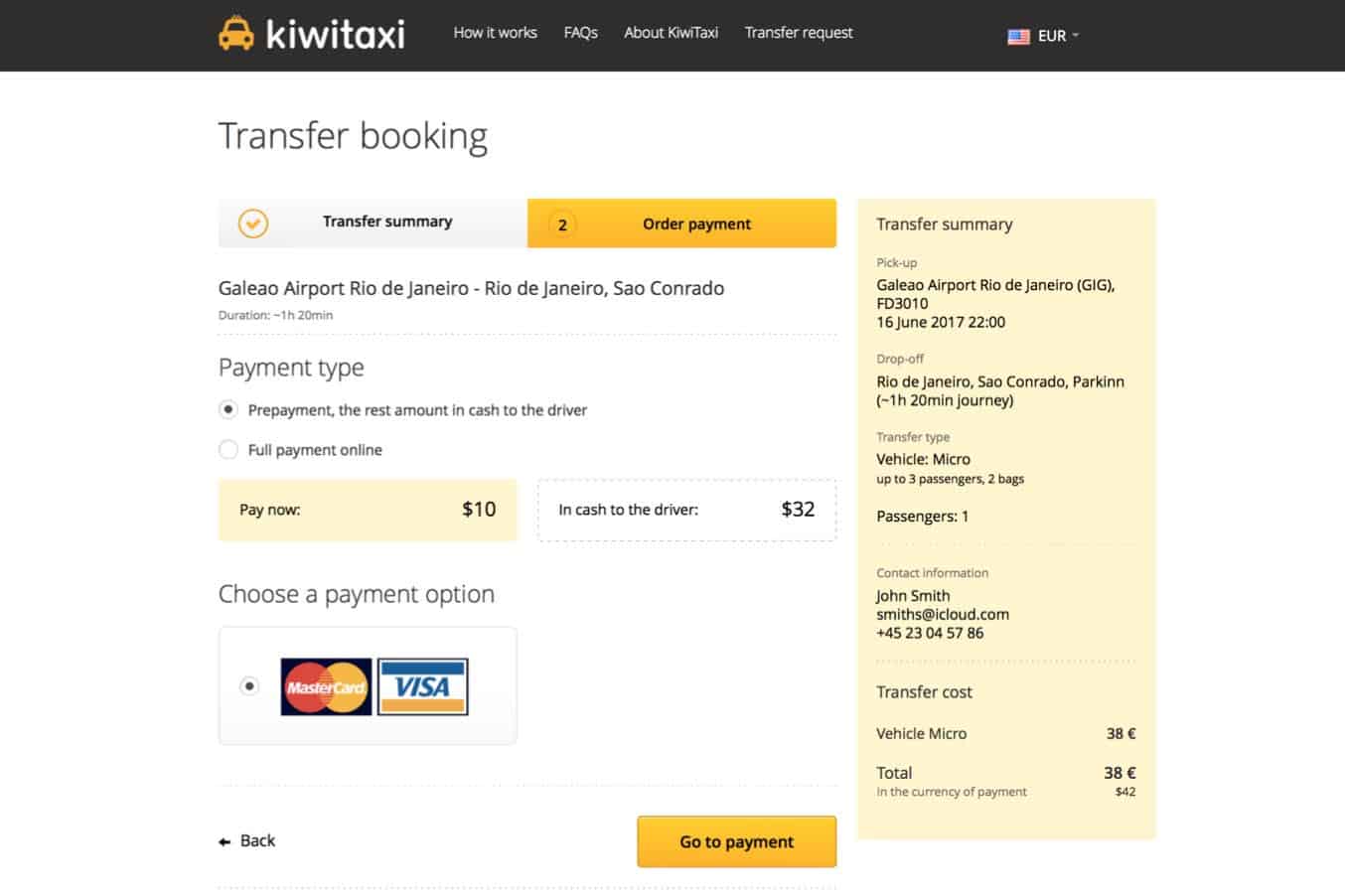The screenshot captures a payment form for KiwiTaxi, prominently displaying their branding and navigation options. At the top, a red and black bar runs horizontally, featuring an orange car logo next to the "KiwiTaxi" name in large white font. The navigation menu includes items such as "How it works," "FAQs about KiwiTaxi," "Transfer request," and an American flag icon with a dropdown currently set to EUR.

The main content area features a large header, "Transfer Booking," followed by several sections. The "Transfer Summary" section is completed, indicated by a check mark. The next section is "To order payment," detailing a transfer from Jelly Isle Airport, Rio de Janeiro to Rio de Janeiro Corrado with a duration of 1 hour and 20 minutes.

Below this, the payment options are displayed. The selected option is "Prepayment," which includes paying a rest amount of $10 online and the remaining $32 in cash to the driver. Another option, "Full Payment Online," is available but not selected.

A prominent yellow button labeled "Pay now $10" is positioned below, followed by the cash amount due to the driver, "$32." Users can choose their payment method from options like Visa and MasterCard, facilitated by a "Go to payment" button.